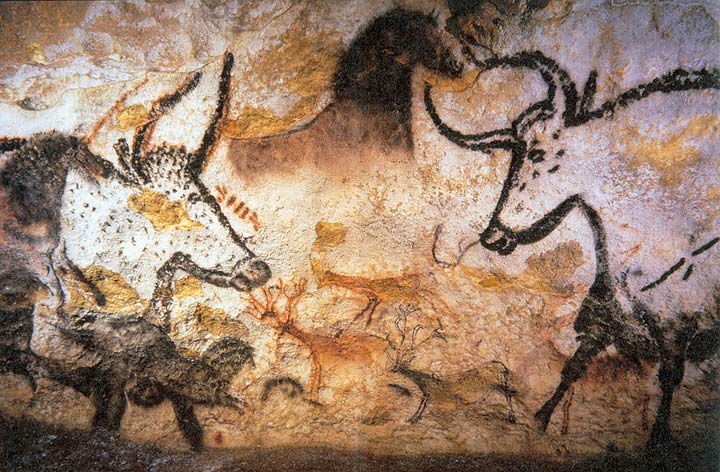This photograph captures a detailed scene of ancient prehistoric cave art, reminiscent of the famous cave paintings in France. Rendered on a textured, lighter rock that resembles parchment paper, the artwork depicts various animals using a limited palette of black, white, and burnt orange or reddish-brown pigments, likely derived from charcoal and natural elements. Dominating the scene are the imposing figures of two aurochs, one on each side, facing off. Both aurochs display distinctive horns and facial markings, created with charcoal.

Above these majestic creatures are rudimentary portrayals of wild horses, also done in dark hues, with some appearing brown. The depiction of the horses evokes a sense of motion and vitality, characteristic of early human attempts to capture the essence of the animal world. Near the bottom and towards the center, faint yet discernible outlines of deer — including a stag and several does — add to the rich tapestry of the mural, rendered in softer brown tones.

This evocative scene blends childlike simplicity with the profound historical significance of early human artistry, resembling caveman etchings. The overlapping images and the earthy, muted color tones convey a timeless narrative from our ancient past.